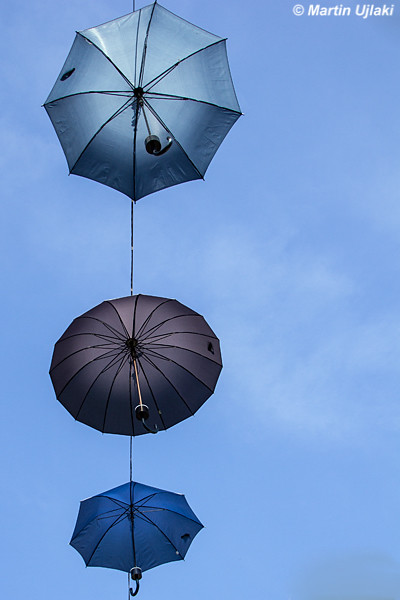In this intriguing image, the viewer's gaze is directed upward towards a bright blue sky dotted with a very thin white cloud. Suspended in the mid-air are three distinctively colored and sized umbrellas, seemingly floating one below the other in a vertical alignment. The topmost umbrella is the largest, featuring a light blue color and an octagonal shape with a black hook handle. It is connected by a thin black string to the middle umbrella, which is black and round, flaunting a brown and black handle. Further down, the smallest and dark blue octagonal umbrella is joined again by a thin line to the one above it. All three umbrellas are open and aligned in a straight line, creating a whimsical and surreal visual. In the upper right-hand corner of the image, the name "Martin Ujlacki" alongside a © symbol appears in white lettering, indicating the copyright holder. Whether this is a real photograph or digitally generated art remains uncertain, adding to the enigmatic charm of the composition.